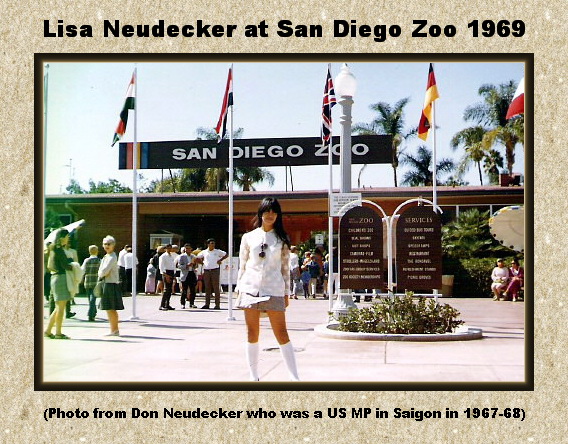The image depicts Lisa Neudecker standing at the entrance of the San Diego Zoo in 1969. The bottom of the photograph bears the caption indicating it was taken by Don Neudecker, who served as a U.S. Military Police officer in Saigon from 1967 to 1968. Lisa, an Asian woman, is dressed in a white jacket, a gray skirt, and white knee-high socks. She has long hair and stands in a relaxed pose amidst a bustling scene. The background reveals a clear blue sky, flags from various countries, and scattered groups of visitors. Concrete medians, palm trees, and outdoor seating areas with white umbrellas also populate the scene. The photo itself is bordered with a light, brown recycled-paper-like frame, lending a vintage feel to this well-preserved memory.